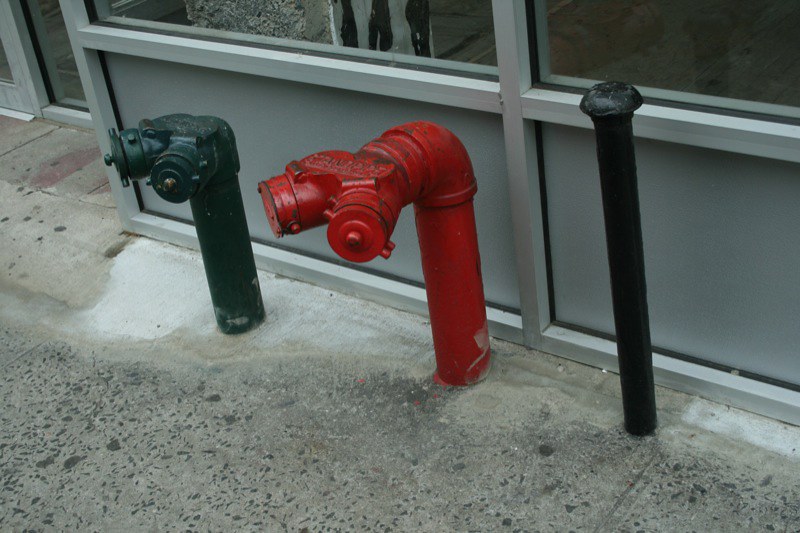The image depicts the exterior of a metal building with a silver-gray facade, characterized by visible construction elements such as joists and panels. The lower section of the building has a row of short windows, with the section of windows above likely clear or mirrored. Below these architectural features, the building's concrete sidewalk is evident, some areas appearing white or unfinished as if recently worked on. Primary subjects in the photograph are three prominent standpipes situated directly in front of the building: on the left stands a black pipe with two fittings for hose connections; the middle pipe is red, also equipped with two fittings, with its structure elbowing out before the outlets; and the pipe on the right is tall, thin, and black, capped with a dome top and devoid of fittings. These pipes, crucial for water hookup, dominate the scene. The beveled building design creates a recess where a door is located on the left side of the frame. The overall color palette features shades of gray, black, red, and some hints of dark green, encapsulating an urban and somewhat industrial ambiance.